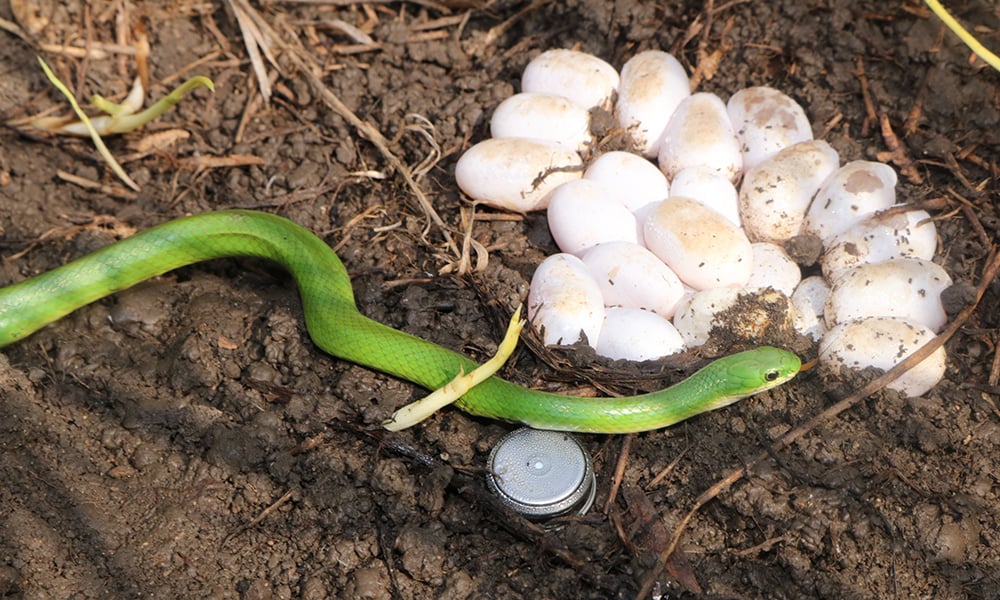In this detailed photograph, taken from a slightly elevated angle, a slender, bright green garden snake with a small head is seen slithering on a moist, muddy ground. The ground is a mix of brown and gray dirt, interspersed with a few twigs, strings, and dried leaves, with sparse green growth visible at the top left corner. The snake, which features black eyes, is approaching a clutch of over a dozen white eggs, significantly larger than one might expect for the snake itself, and slightly smaller than chicken eggs. These eggs lie on the right side of the image, their surfaces dirtied from their environment. In the center foreground, partially beneath the snake, there is a round, metallic object embedded in the ground, likely a garden sprinkler, hinting at a potential garden setting. Additionally, a piece of plastic litter is visible below the snake, adding a touch of realism to this intriguing scene of nature.